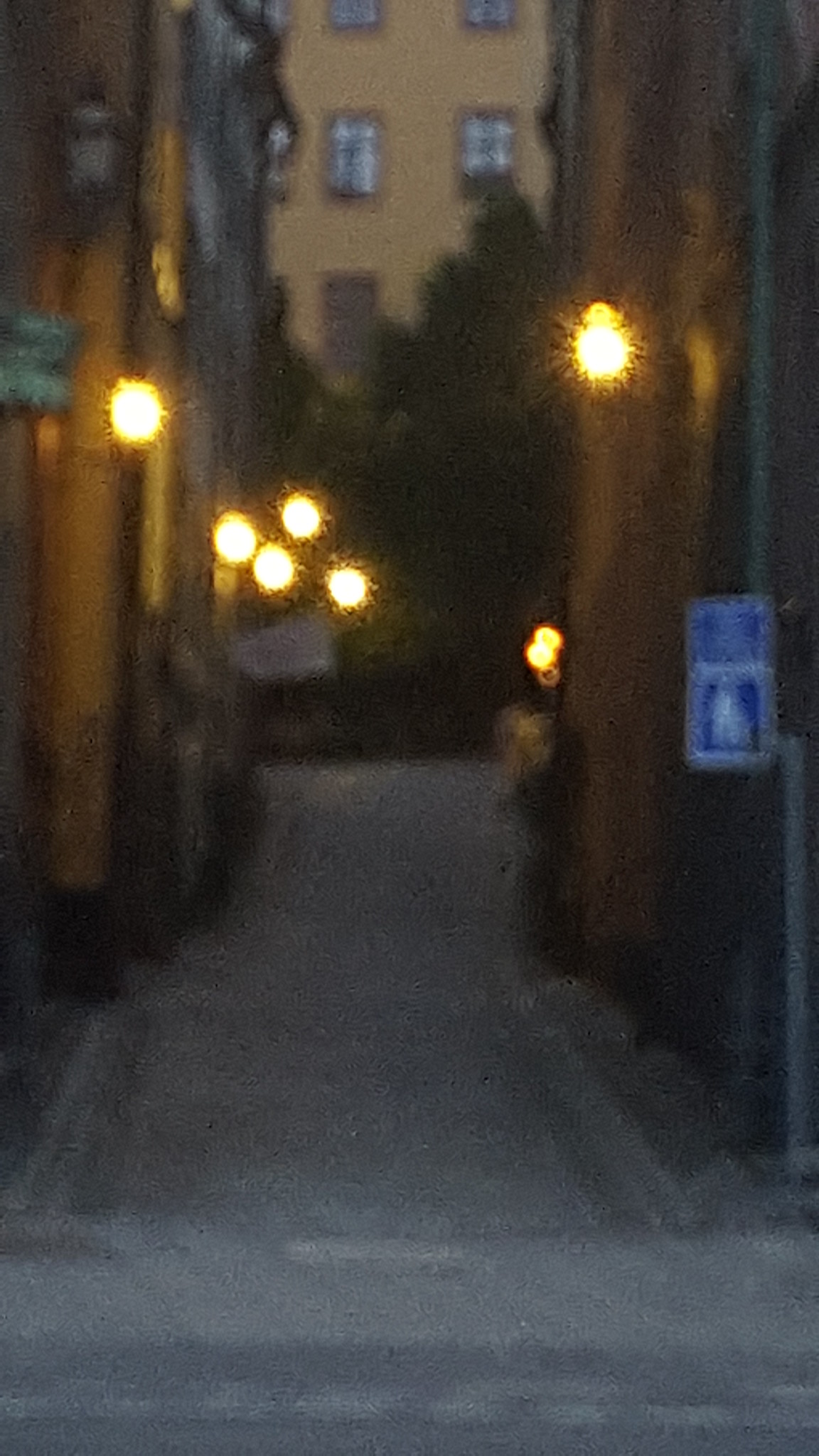This blurry vertical photograph captures a street scene taken at dusk in what appears to be a charming, walkable European city. The image shows a narrow alleyway flanked by tall, older buildings with brick-like facades in medium brown hues, accentuated by darker trims. The buildings are adorned with illuminated street lights that cast a golden glow across the scene. Through the alleyway, a large apartment building with light-colored window shades is visible, encompassing the rear of the image. A tall, green tree stands prominently in front of this building, adding some natural contrast to the urban environment. 

In the foreground, the gray pavement of the street and sidewalk is visible. On the right-hand side of the image, there is a street light post with two distinct blue signs featuring white figures, suggesting pedestrian activity or signaling a crosswalk. The background reveals several small, glowing lights stringing across the alley, enhancing the cozy and inviting atmosphere. Despite the distortion, the city's inviting character is palpable, enriched by the contrast between the bustling lights and the serene twilight sky.